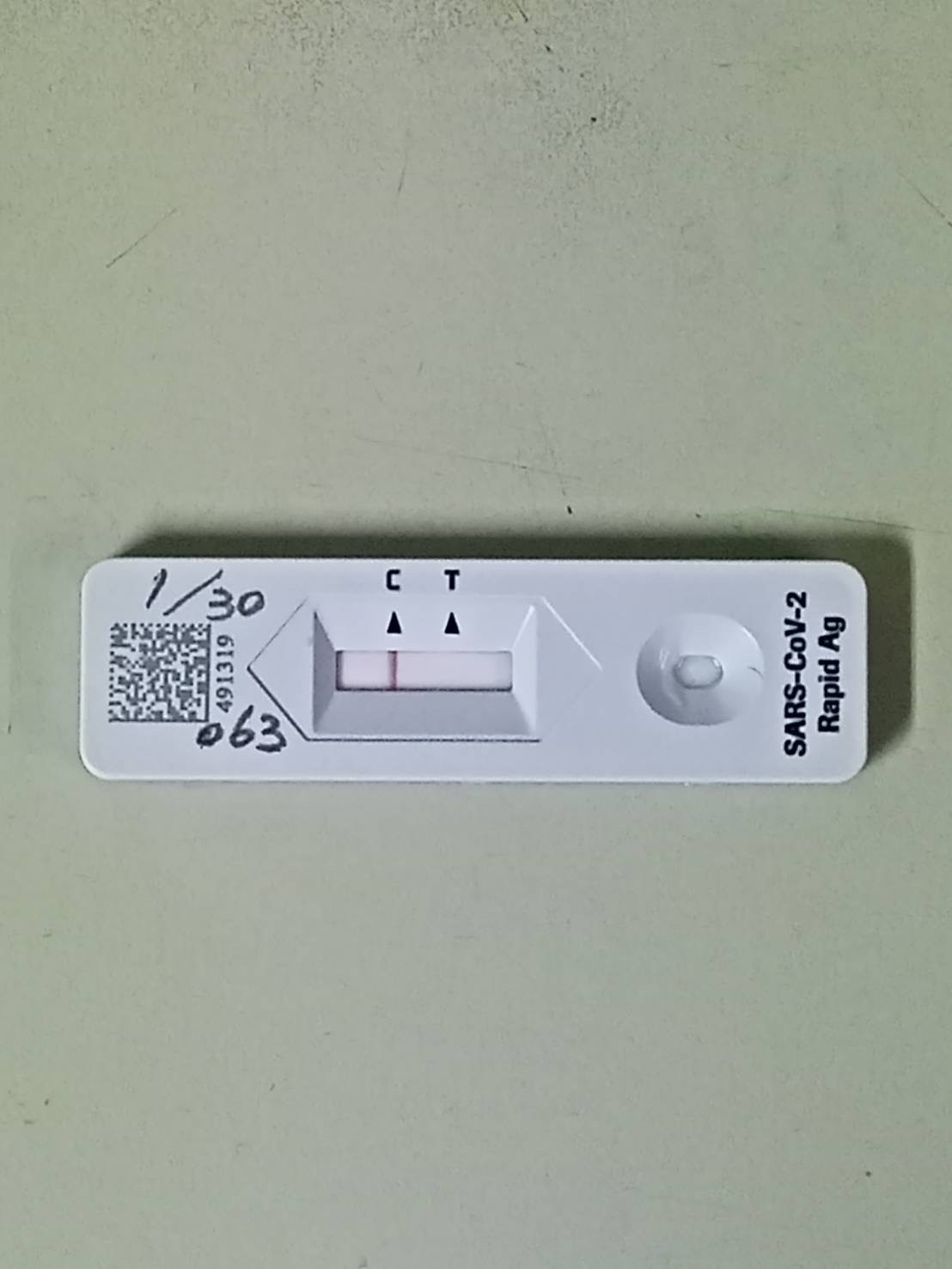The photograph features a COVID-19 test device prominently displayed against a completely gray background. The testing apparatus occupies approximately 85 percent of the image, casting a shadow that extends upward and to the right.

The COVID-19 test is primarily white with black lettering and various inscriptions. Starting from the left side, there is a QR code. Above the QR code, the text "1/30" is printed, while "063" is found below it. Adjacent to the QR code, the sequence "491319" is inscribed. 

Towards the center of the test, there is a small window outlined by an upward-pointing arrow labeled "C" and another arrow pointing to "T." Inside the window, a vertical line is visible against a white background, aligning with the arrow and the letter "C."

On the right-hand side of the test, there is an oval containing a smaller gray oval at its center. The rightmost edge of the device features the text "SARS/COV-2 Rapid AG."

Overall, the image provides a detailed view of the COVID-19 test device, highlighting its various components and labeling.